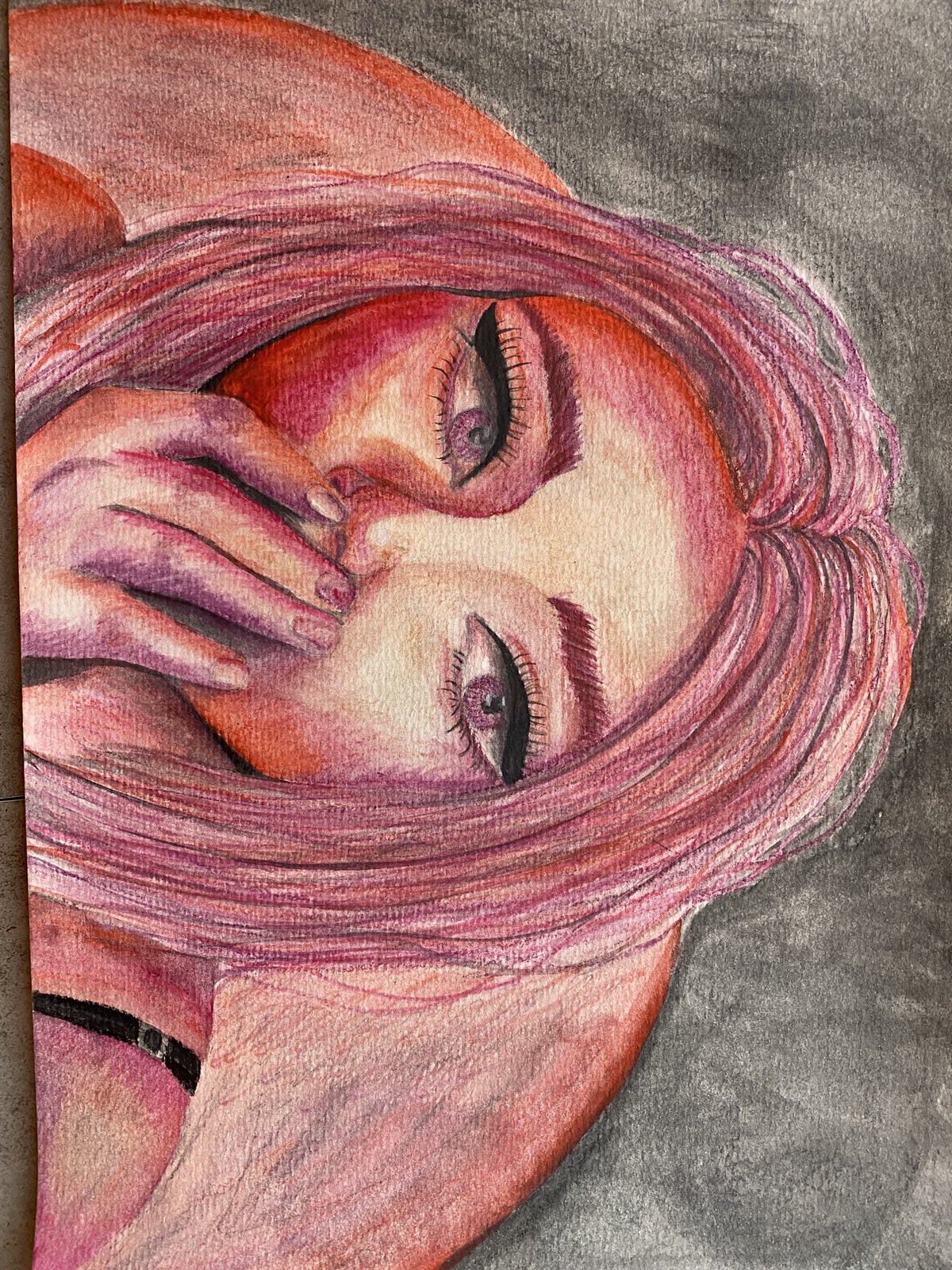This image is a sideways view of a detailed sketch, seemingly created with colored pencils. The artwork features a close-up of a woman, focusing primarily on her head and the upper portion of her shoulders. The woman has one hand raised, covering her mouth and partially obscuring her expression. Her most striking features are her large, violet-blue eyes, accentuated with heavy upper lid eyeliner and well-defined eyebrows. The facial contours are rounded and portrayed with vibrant red and pink tones, matching the hues in her straight hair that falls past her shoulders. The entire composition is set against a muted gray background, allowing the vivid colors of her hair and face to stand out.